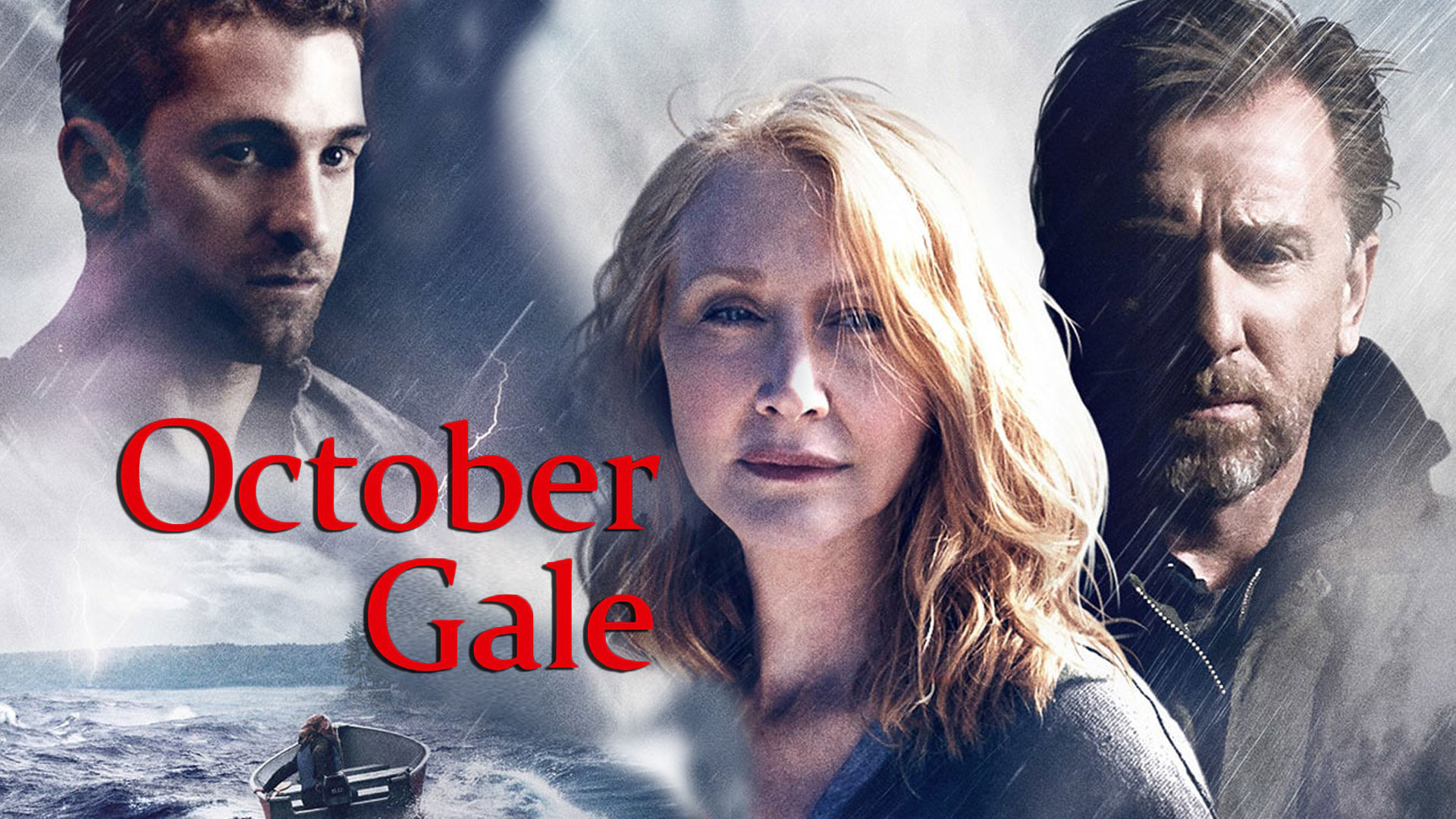This promotional poster for the film "October Gale" features a collection of color photographs combined with graphic design and typography. The image is a landscape-oriented collage showcasing three central characters against a stormy backdrop with lightning bolts.

At the forefront and slightly to the right, actress Patricia Clarkson is depicted from the shoulders up, gazing directly at the viewer with a concerned expression. She has shoulder-length reddish-brown (or blonde) hair. To Patricia's right stands Tim Roth, identifiable by his dark hair, salt-and-pepper beard, and black jacket. He appears to be gazing downward with a subtle frown.

On the left side of the poster, a third man with dark hair and a scruffy beard is positioned. He seems to be wrapped in a blanket or similar garment and is looking towards the center of the image.

The background evokes a sense of stormy weather, with a dramatic sky filled with dark clouds and lightning. In the bottom left corner, there's a smaller inset image of a single person in a small boat navigating rough waters, heading towards a storm with plants and trees visible on the shore.

The movie title, "October Gale," is prominently displayed in red letters towards the bottom left of the poster, with "October" positioned over "Gale" and aligned on the right side of the typography.